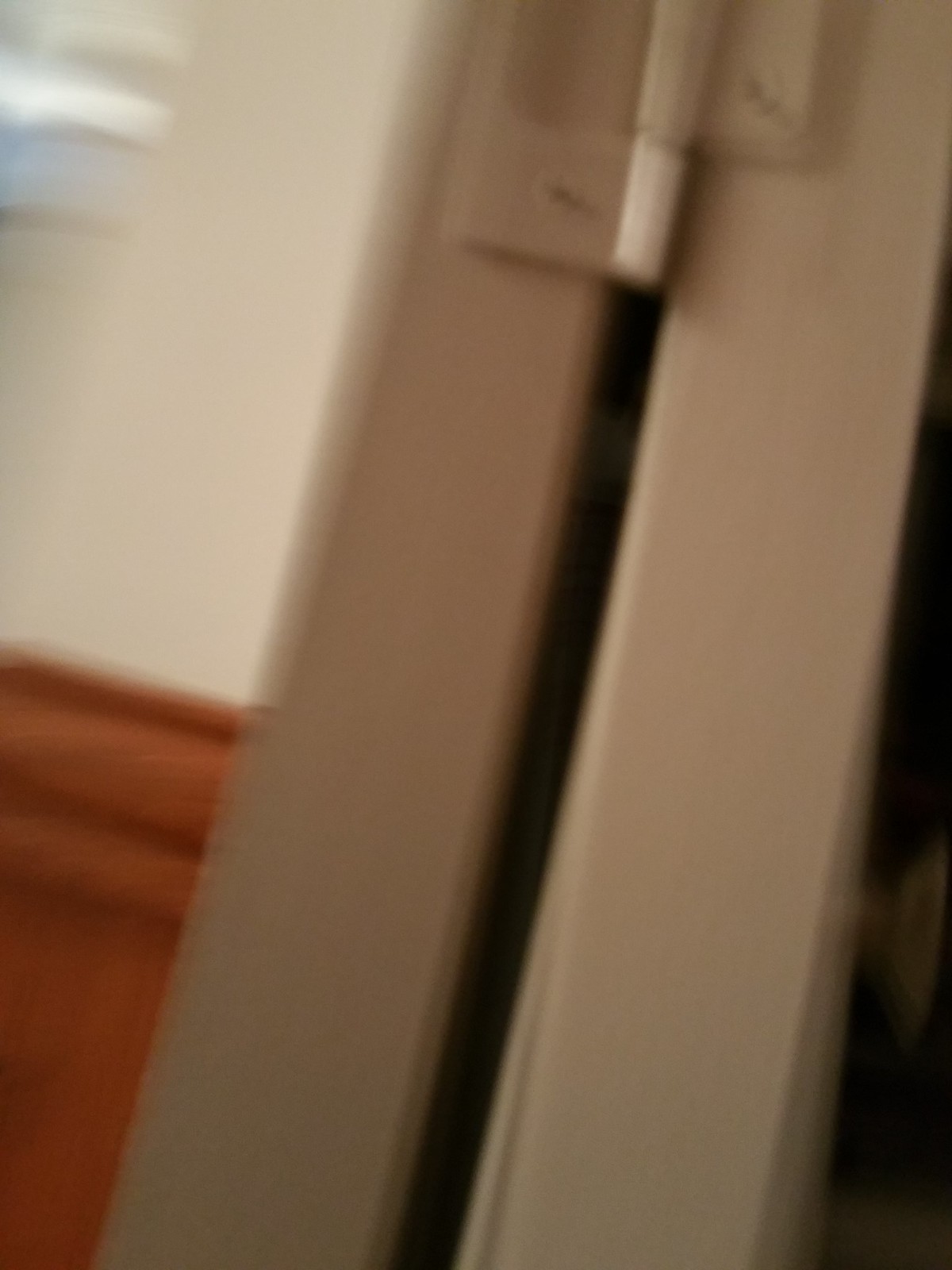This photograph, though blurry and seemingly accidental, shows a close-up view of an interior scene. The main focus is on a cream-colored hinge attached to two long, cream-colored rectangular objects appearing to be door panels or parts of a folding door, positioned slightly apart, revealing a notable gap. The hinge is visible along with two screws, suggesting it’s meant for something that folds or swings open, likely a closet or cupboard door. To the left, there's a section of the image showing a light cream or off-white surface, possibly a wall, and a brown area with decorative trim towards the top, which may be an adjacent wall or furniture piece. Despite the poor quality and blur of the photo, these elements come together to suggest an indoor location, capturing parts of a folding door or cabinet amidst its surroundings.